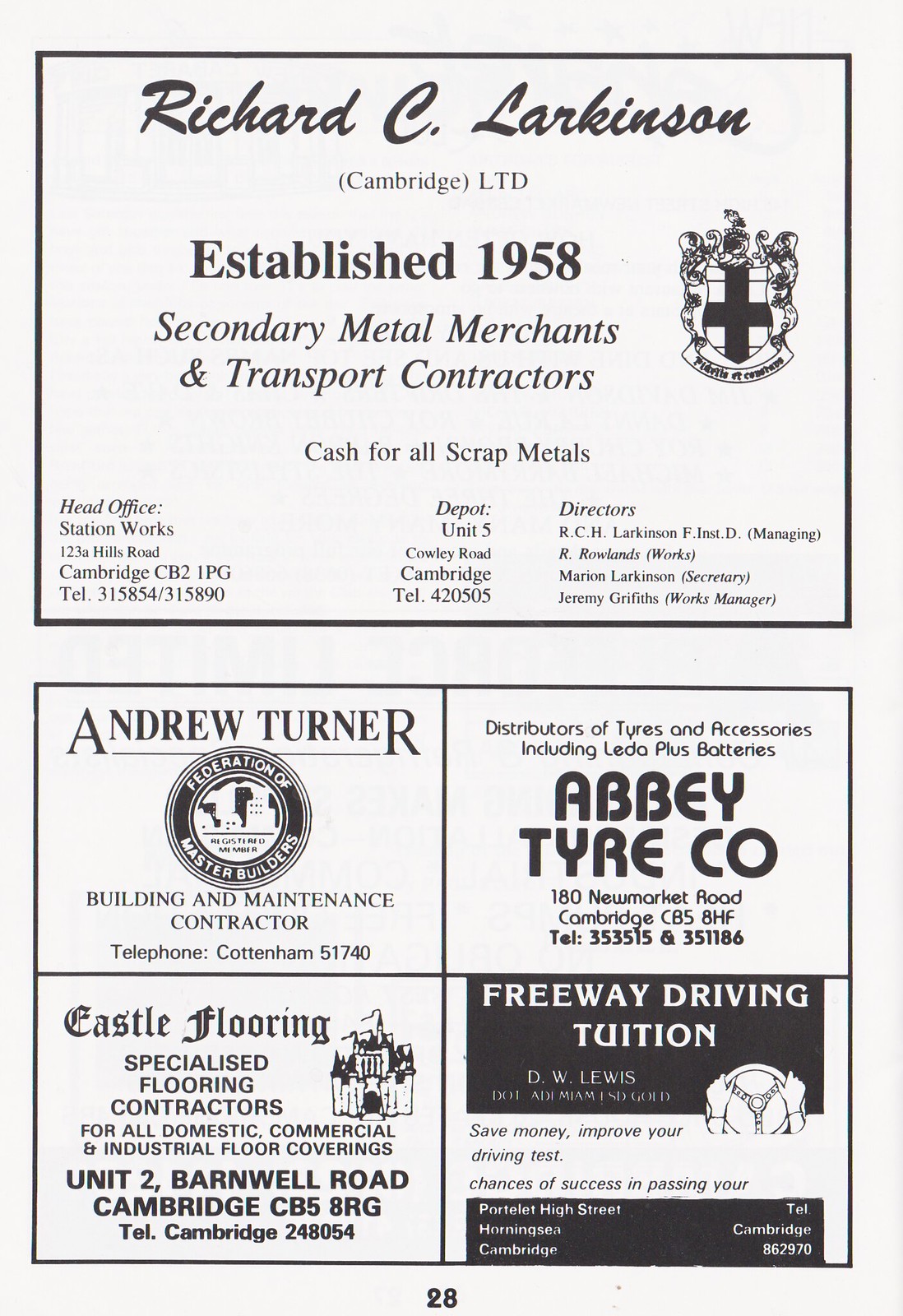This is a scan from an old program booklet, likely from a magazine or sports event. The page features five black-and-white advertisements. At the top, the largest ad, taking up half the page, is for Richard C. Larkinson Cambridge LTD, established in 1958. It provides services as secondary metal merchants and transport contractors, offering cash for all scrap metals. This ad includes information about the head office, depot, directors, and prominently features a family crest on the right side.

Below are four smaller advertisements arranged in a grid. The top left ad is for Andrew Turner, a Federation of Master Builders member, offering building and maintenance contractor services. The top right ad is for Abbey Tire Company, highlighting their distribution of tires and accessories, including Lida Plus Batteries. The bottom left ad is for Castle Flooring, specialized flooring contractors. The bottom right ad is for Freeway Driving Tuition, offering driving lessons. All advertisements provide contact numbers and addresses, maintaining the monochromatic theme of the page.